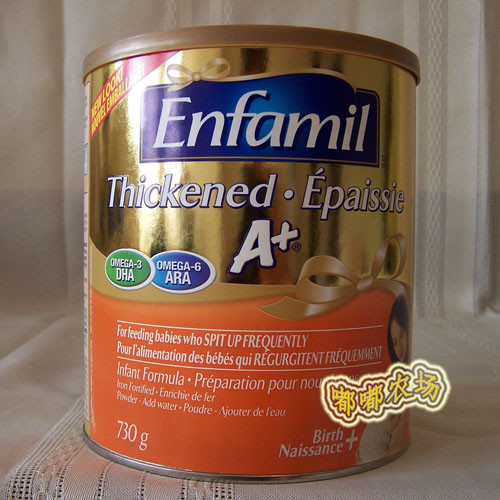This photograph features a cylindrical can of Enfamil baby formula prominently displayed on a white cloth backdrop. The can is adorned with a gold lid and features a label that transitions from gold at the top to a pinkish-salmon hue towards the bottom. The brand name "Enfamil" is prominently displayed on a blue banner at the top of the can in white letters, with a gold bow accentuating the banner. Below this, the text "Thickened A+, Omega-3 DHA" is written in both English and French, indicating that the formula is designed for feeding babies who spit up frequently. The can also includes additional information like "Infant formula, iron fortified, powder, add water, 730 grams, birth plus." Scattered green and blue circles highlight some ingredients on the label, enhancing its visual appeal. Furthermore, Chinese text, in yellow with a cream-colored outline, is superimposed over the image near the bottom right, partially obscuring a depiction of a woman with a downward gaze.